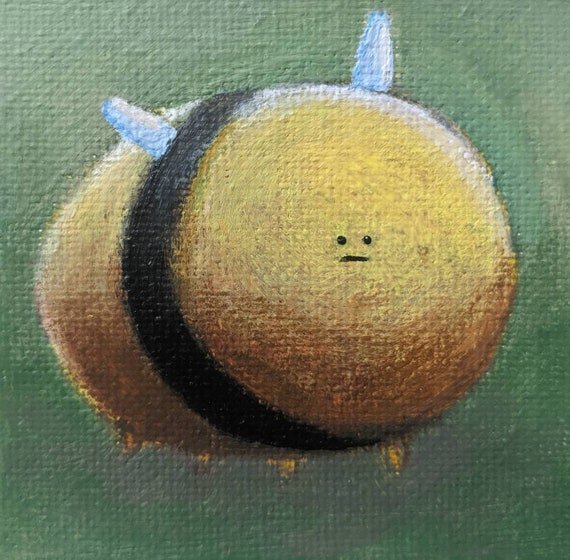This painting features an extremely stylized and whimsical depiction of a bumblebee that evokes a children's book character. Set against a green canvas background, the bee dominates the entire frame with its exaggerated, oblong body shape that resembles a minion, further enhanced by its vibrant yellow hue mixed with hints of burnt orange. The bee sports two tiny black dots for eyes and a simple straight black line for a mouth, giving it a frumpy and possibly unhappy expression. A single black stripe encircles its midsection, while its four nubby little yellow legs protrude beneath its large, bloated form. Additionally, the bee has two white antennae standing up from its head and some subtle white shading at the top of its body. Despite its charmingly simplistic and exaggerated design, the overall effect is more caricature than realistic, as if illustrated by Dr. Seuss.